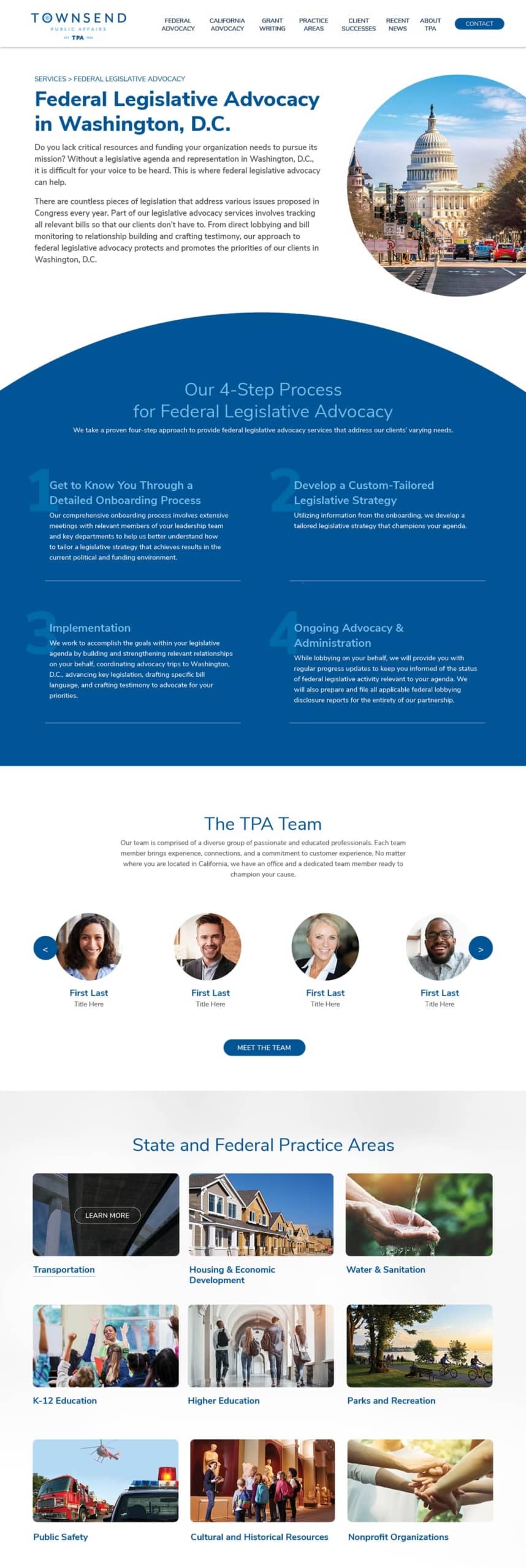The image displays the Townsend Public Affairs (TPA) website, but it has been stretched horizontally, making the text difficult to read. At the top of the page, there is a navigation menu featuring options such as Federal Advocacy, California Advocacy, Grant Writing, Practice Area, Client Success, and Recent News about TPA. A prominent blue button labeled "Contact" is also visible in this section.

Beneath the navigation menu, a horizontal line separates the header from the content below. The content area begins with a section titled "Services," focusing specifically on "Federal Legislative Advocacy," which is emphasized with enlarged text. 

The text elaborates on the challenges organizations face in securing essential resources and funding necessary to advance their missions without a solid legislative agenda and representation in Washington, D.C. It highlights the importance of federal legislative advocacy in amplifying an organization's voice amidst numerous legislative issues considered by Congress each year.

The description proceeds to explain TPA's comprehensive approach to federal legislative advocacy, which includes tracking relevant bills, direct lobbying, bill monitoring, relationship building, and crafting testimony. These efforts ensure the protection and promotion of client priorities in Washington, D.C.

The section concludes by mentioning a "four-step process for federal legislative advocacy," suggesting a structured methodology employed by TPA to achieve successful outcomes for their clients.